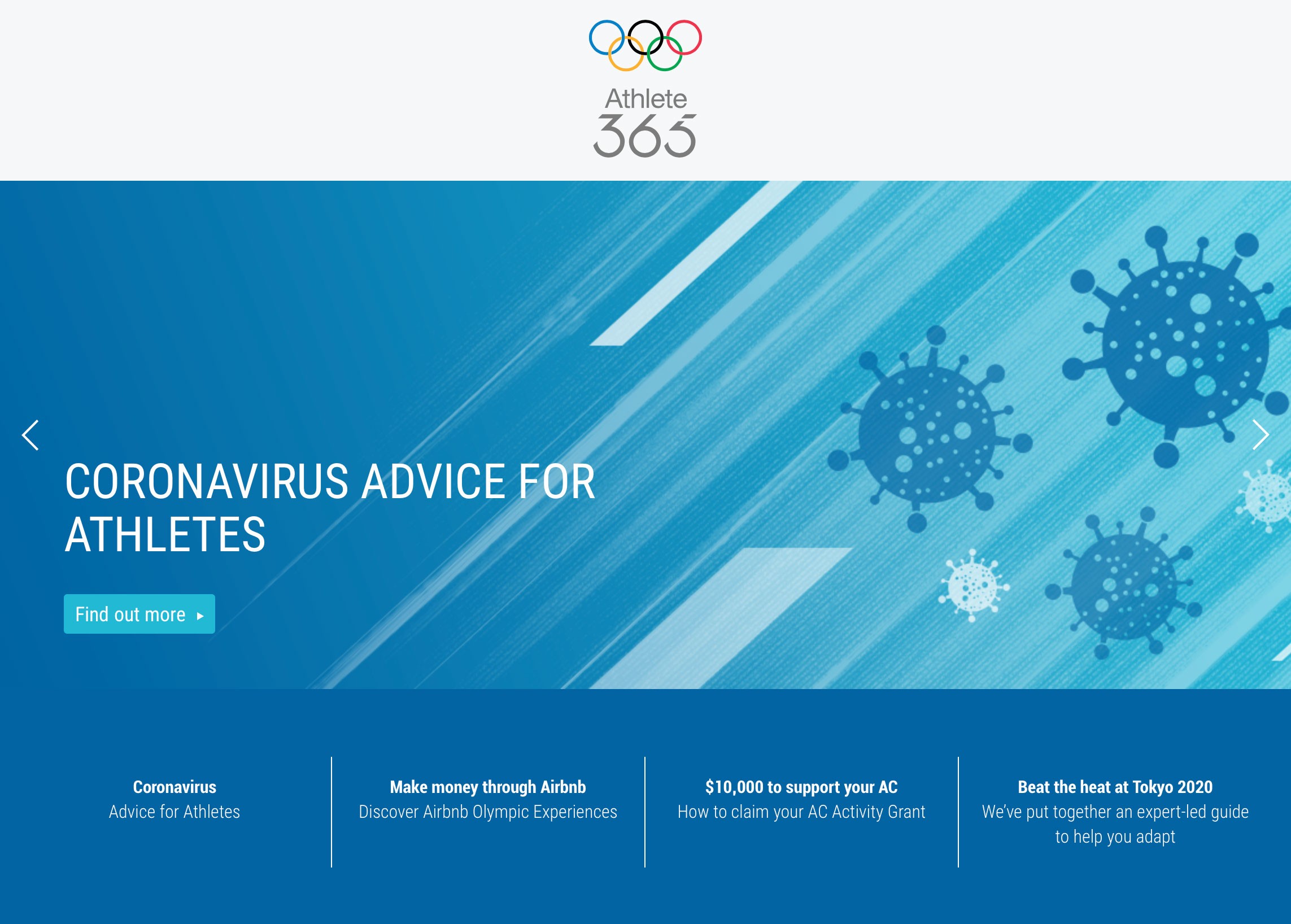This image is a screenshot, with a horizontal orientation. At the top, against a very off-white background, prominently displayed in the center is the Olympic icon featuring five interlocked rings in rainbow colors: blue, purple, and red in the top row, and yellow and green in the bottom row. Below the icon, in gray text, is the phrase "Athlete 365." Underneath that, there is a blue rectangular box with white text stating "Coronavirus advice for athletes." A blue action button underneath the text reads "Find out more."

Near the bottom of the image, a dark blue footer spans the width of the screen. From left to right, the footer displays different topics: "Coronavirus advice for athletes," "Make money through Airbnb," "Discover Airbnb Olympic experiences," "$10,000 to support your AC and then beat the heat at Tokyo 2020." Lastly, it mentions, "We've put together an expert-led guide to help you adapt."